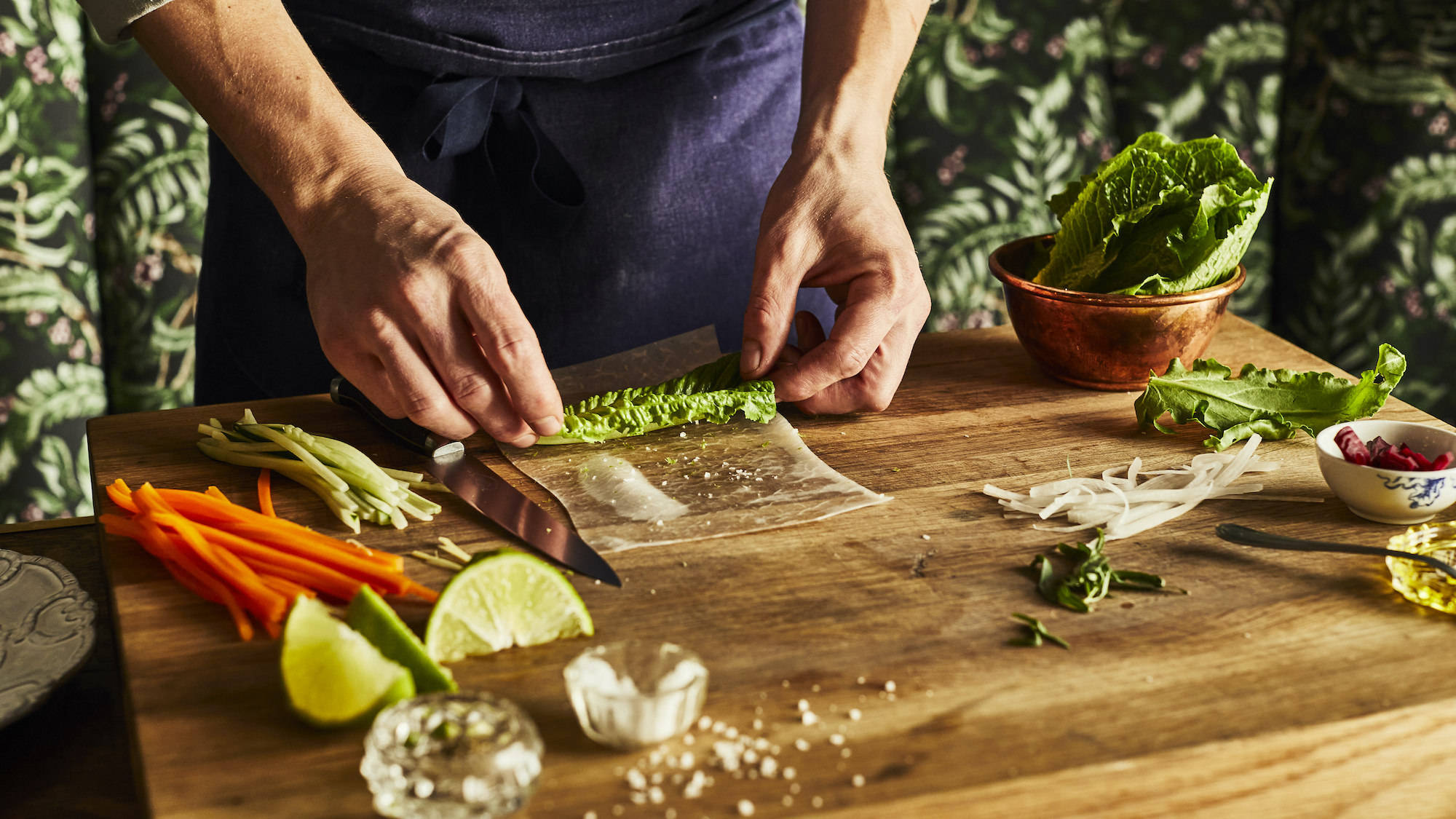In the image, a person is meticulously preparing vegetables on a wooden cutting board. The individual is dressed in blue jeans overalls and is shirtless, visible from the waist to the top of the thighs. The background is adorned with green curtains that have a floral or shrub-like pattern, giving the impression of lush greenery or trees.

The person's hands are busy at work, with a very sharp knife prominently placed on the wooden cutting board. To the left side of the image, the person is seen organizing various ingredients. There are eight to ten peeled strips of carrots, a lime cut into three pieces, several scallions, and some green leafy vegetables that appear to be romaine lettuce.

A brown bowl on the table contains additional long leaves of romaine lettuce, while more of the same lettuce is spread across the surface. Nearby, something that might resemble peppers is placed among the assortment. Additionally, there is a white bowl containing red berries or a similar red item, though it is not entirely clear. A spoon rests on a yellow plate, completing the scene of a well-prepared and organized cooking space.